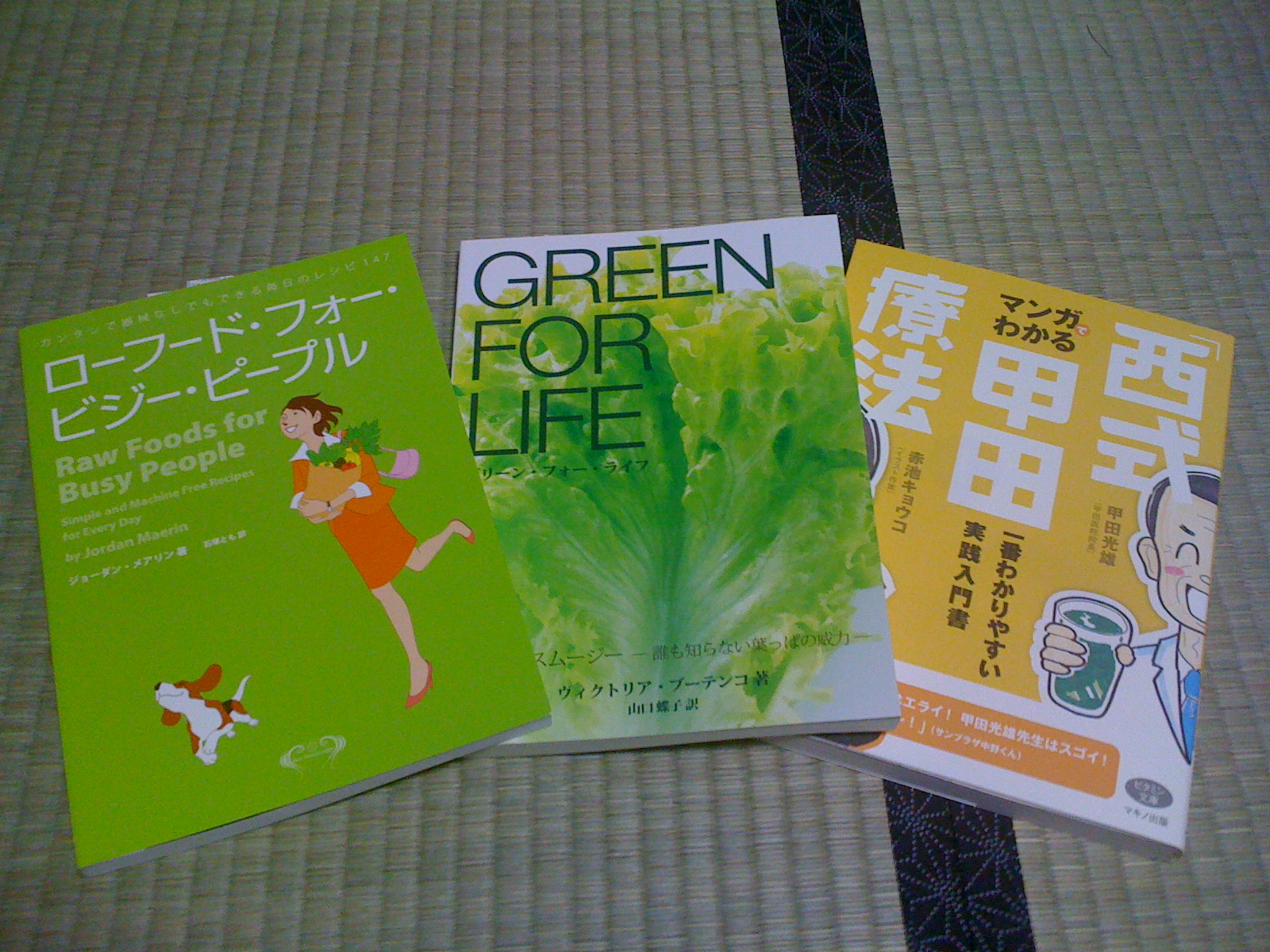This image features three paperback books arranged in a fanned-out manner on a pale beige, woven mat with a black stripe running vertically. The book on the left has a lime green cover with Chinese characters at the top, and beneath them, the English title "Raw Foods For Busy People." It depicts a cartoon woman in a red dress, brown hair, and red shoes, carrying a bag of groceries, accompanied by a small brown and white dog with its ears flapping. The center book, with a white, lime green, and medium green background, prominently displays the title "Green for Life" in large dark green print, alongside a large image of a green leaf of romaine lettuce and additional Chinese text. The book on the right features a yellow and white cover, with more Chinese characters and a cartoon character of a man in a white lab coat and blue tie, holding a glass filled with green liquid. The books stand out against the intricate pattern of the background mat, which adds a textured, homey feel to the composition.